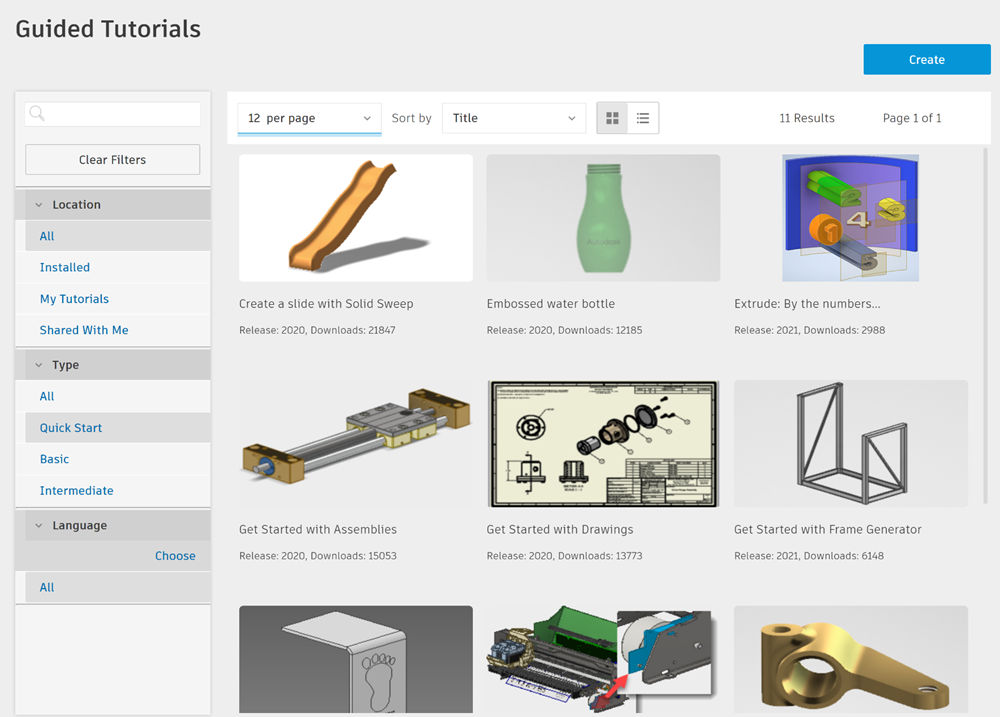The screenshot depicts a webpage dedicated to Guided Tutorials. The page features a clean design, characterized by a light gray background and black font for enhanced readability. At the top-left corner, the title "Guided Tutorials" is prominently displayed. Directly beneath the title, users will find a search entry box which allows them to set specific filters.

Beneath the search entry box, there are options to select the location, type of tutorials, and the available languages. This filtering functionality is neatly organized on the far left side of the page.

The central part of the webpage showcases a variety of tutorials. Presently, six tutorials are clearly listed with detailed titles, while three additional tutorials at the bottom merely display images without accompanying descriptions. The tutorials include:
1. **Creating a Slide**
2. **Creating an Embossed Water Bottle**
3. **Creating an Object with Numbered Descriptions**
4. **Getting Started with Assembly**
5. **Getting Started with Drawings**
6. **Getting Started with a Frame Generator**

The webpage is designed to display up to 12 tutorials per page, although in this particular screenshot, only nine are visible. Of these nine, six tutorials have visible titles, while the remaining three are identified solely by their images. This structured layout aids users in easily navigating through the tutorial options and finding the specific guides they need.